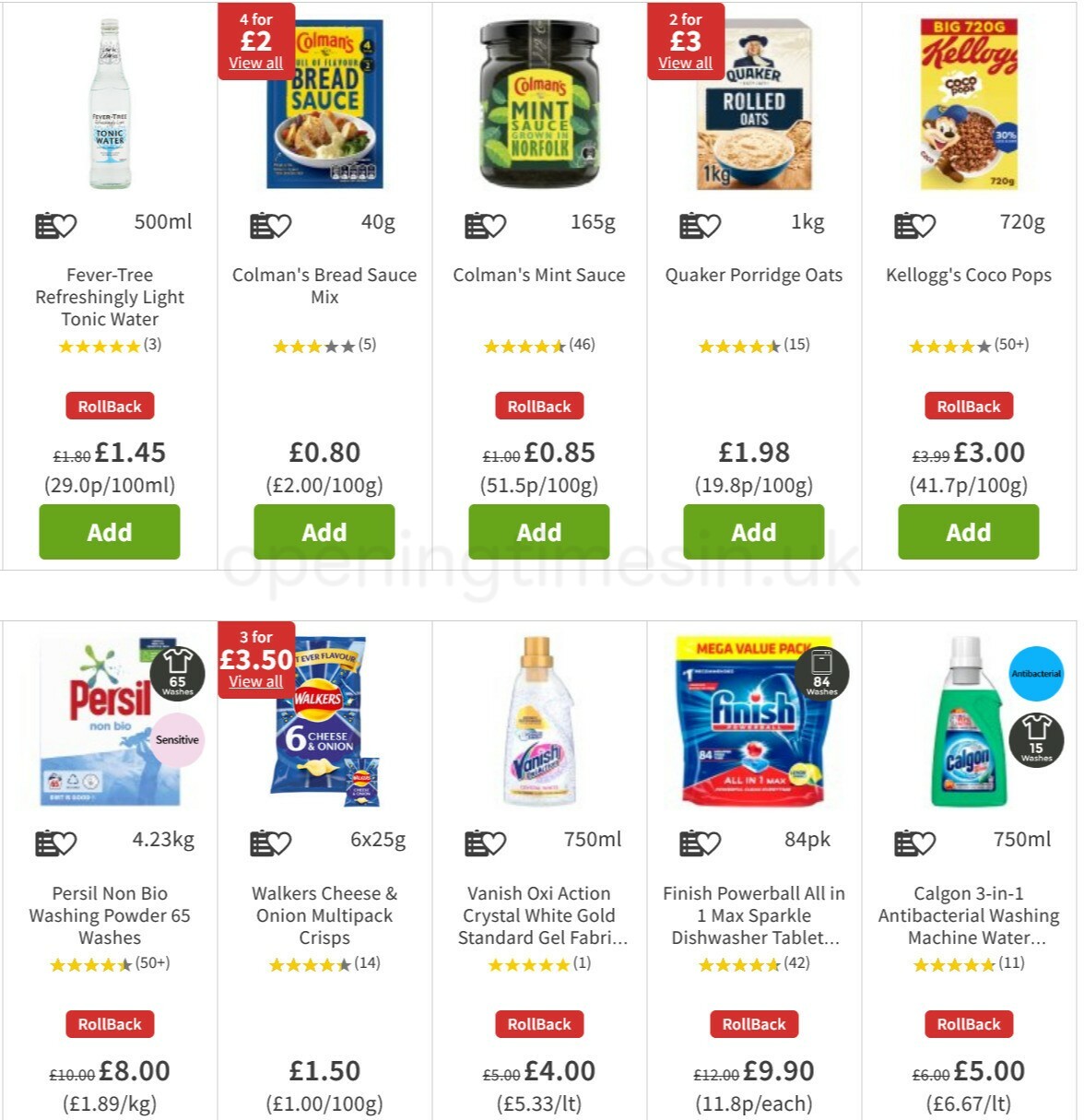The image showcases a selection of various products available for purchase. The featured items include:

1. Fevertree Refreshingly Light Tonic Water
2. Coleman's Bread Sauce Mix
3. Coleman's Mint Sauce
4. Quaker Porridge Oats
5. Kellogg's Cocoa Pops
6. Persil Non-Bio Washing Powder (65 Washes)
7. Walker's Cheese and Onion Multi-Pack Crisps
8. Vanish Oxy Action Crystal White Gold Standard Gel Fabric
9. Finish Powerball All-in-One Max Sparkle Dishwasher Tablets
10. Calgon 3-in-1 Antibacterial Washing Machine Water

A notable aspect of the image is the presence of "Add" buttons beneath the first five products, while the remaining items lack these buttons, likely due to the image being edited or scrubbed.

Several products are highlighted with special offers:
- **Coleman's Bread Sauce Mix:** "Four for £2" with a "View All" link.
- **Quaker Porridge Oats:** "Two for £3" with a "View All" link.
- **Walker's Cheese and Onion Multi-Pack Crisps:** "Buy Three for £3.50" with a "View All" link.

Interestingly, the only products without rollback indications are the Coleman's Bread Sauce Mix, Walker's Cheese and Onion Multi-Pack Crisps, and Quaker Porridge Oats. All other items feature a red "Rollback" button beneath them, signaling a potential price reduction or promotion.

The detailed presentation and promotional details make this an enticing display for potential buyers, highlighting both availability and special offers on selected items.